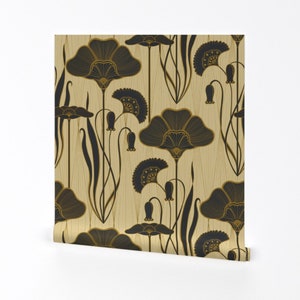The image is a small, square artwork set against a very light gray background, presented at a slight angle, giving it a perspective effect similar to a product photo. This possibly textile or painting features a central, creamy beige to light sandalwood background with intricate floral designs. The floral patterns encompass various shades of blacks, dark greens, and golds. Scattered throughout the cream-colored background, the artwork displays different flower shapes and stems. Some flowers have drooping bulbs resembling tulips, while others are side-view, fan-shaped resembling semi-circles. The centerpiece is marked by stems with long, winding lines, some stretching diagonally across the textile. One prominent stem, winding from left to down and up to the right, stands out in a darker shade in the middle. The floral design is rich in detail with string-like stems and umbrella-shaped tops, offering a harmonious blend that repeats and complements the sophisticated pattern. The image contains no people or text, focusing purely on the serene floral artwork.